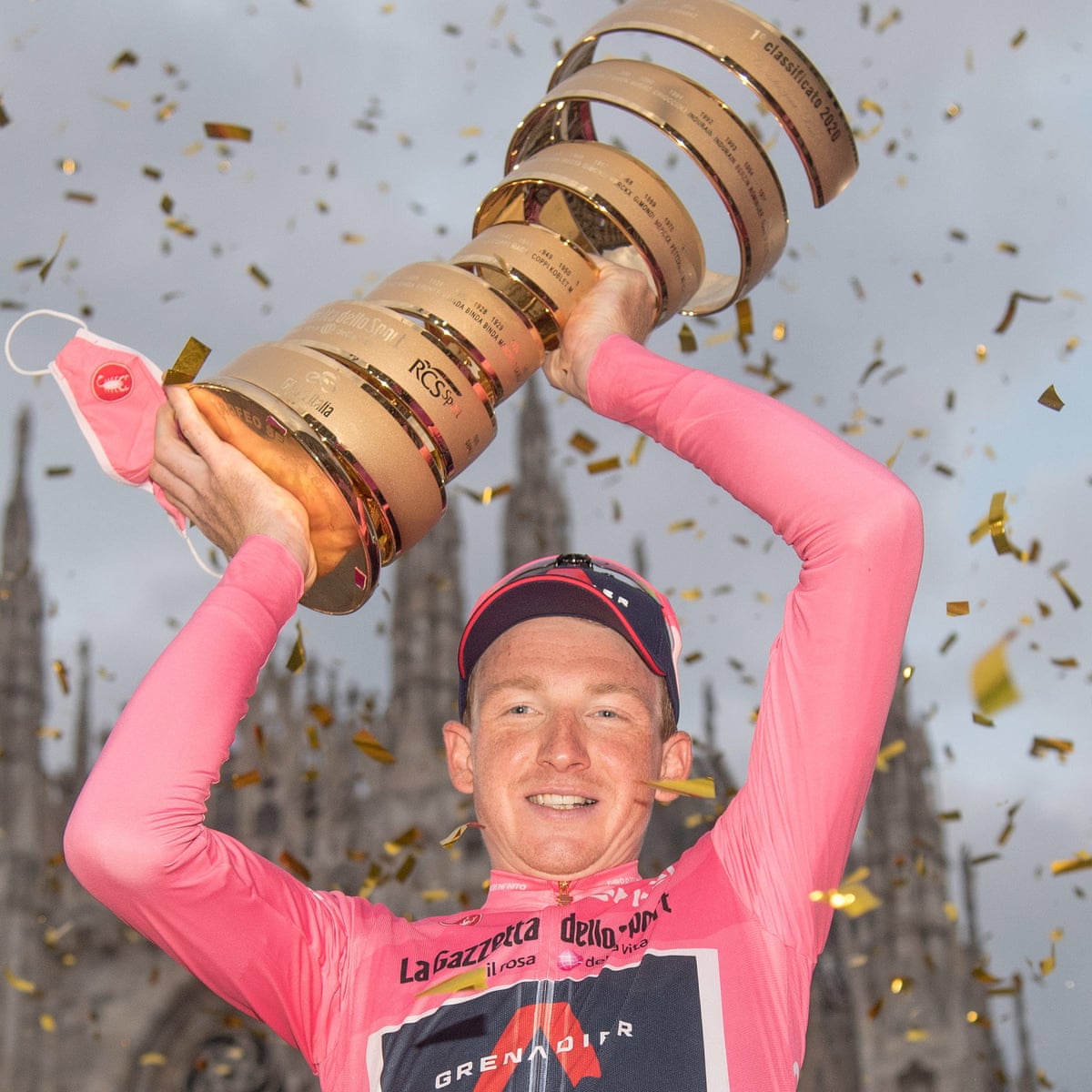In the photograph, a smiling white male athlete with a red and black baseball cap is seen triumphantly holding a large, gold, spiral trophy above his head. The trophy, adorned with text such as "Classificato 2020" and "RCS SP," features a wide base that narrows upward through several loops before expanding again. He is dressed in a long-sleeved, skin-tight pink bodysuit starting at his neck and extending to his wrists. Prominently displayed on the bodysuit's chest are the words "La Gazzetta dello Sport," an Italian newspaper, and a black square with the word "Grenadier" inscribed over an inverted red V. The background is animated with raining gold confetti and a blurry view of a large, brown cathedral-like building, suggesting the location might be Italy. The athlete exudes joy, embodying the victorious moment captured in the celebratory atmosphere.